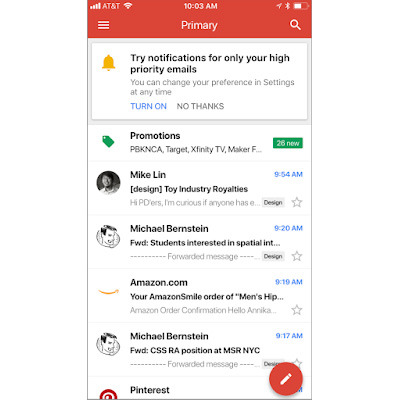This is a detailed screenshot of a cell phone screen displaying a Gmail interface. At the top of the screen, the status bar indicates the time as 10:03 AM. The battery icon shows a charge level of approximately 75%. Bluetooth and location services are active, and the device is connected to Wi-Fi. Additionally, the AT&T network has full reception with four out of four bars. 

Below the status bar, there are three horizontal lines indicating a menu dropdown on the left, the word "Primary" in the middle, and a search icon represented by a magnifying glass on the right. Next is a notification prompt suggesting, "Try notifications for only your high priority emails." The user has the options to change preferences and settings at any time, with buttons labeled "Turn on" and "No thanks", accompanied by a yellow bell icon to the left.

Proceeding further down, the screen displays the "Promotions" folder with email previews starting from "pbknca," "Target," "Xfinity," "TV maker," indicating there are 26 new emails. The first email listed is from Mike Lynn, with the subject "Design, Toy Industry Royalties" and a fragment, "Hi pdrs, I'm curious if anyone has..." received at 9:54 AM. Following that is an email from Michael Bernstein with the subject "Forward students interested in spatial" received at 9:20 AM. Further emails are from amazon.com, another from Michael Bernstein, and lastly, from Pinterest.